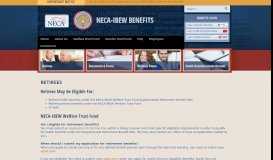Here is a detailed, cleaned-up caption for the described image:

---

The image depicts a miniature version of a website, highlighted by a series of colored bands. At the top, there is a thin yellow band followed by a slightly thicker blue band featuring a darker blue center. Within this blue section, there is a square logo with the letters "N-E-C-A" and a round crest logo that mentions "N-A-C-A" benefits. Below this is a red band showcasing two small images; the first image contains what appears to be two individuals, likely a woman and a man with a beard. The second image is indiscernible. Continuing downward, there is another blue band with white text, then a third image displaying a woman and a man’s head. Beneath this is yet another blue band with white text, followed by a fourth image showing open books or notebooks. This image is also flanked by red bands. Finally, there is a beige band at the bottom with multiple paragraphs of black text, featuring larger headings and smaller, hard-to-read paragraph text.